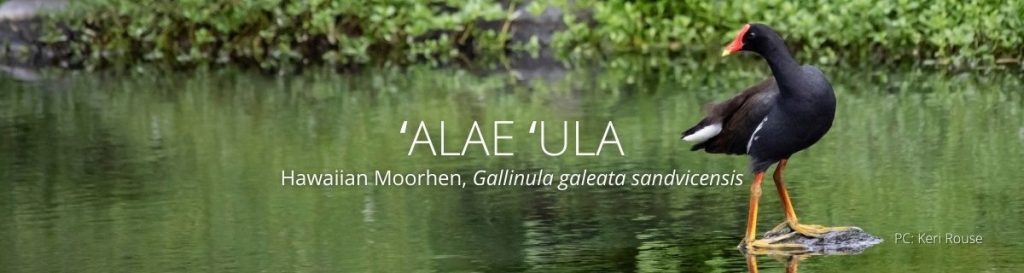The image is a wide, panoramic advertisement or poster that primarily features a serene lake. Dominating the frame is a tranquil body of water, bordered at the top by a dense row of lush shrubs and bushes. The forefront of the image captures a striking black bird, similar in appearance to a duck but with distinctive features: an orange-red patch on its forehead transitioning into its beak, predominantly black feathers accented by a small patch of white on its wings, and long, yellowish-orange legs standing on what seems to be a rock or lily pad in the water.

The bird is positioned towards the right side of the image, with its body facing right and its head turned back to the left. Overlaying the water in the middle of the image is bold white text featuring the name "(Alaeula)" in large letters. Below this, in smaller font, the text reads "Hawaiian Moorhen, Gallinula Sandvicensis," indicating the common and scientific names of the bird. Additional faint white writing, difficult to decipher, is located in the bottom right corner, likely attributing the photograph to "P.C. Kerry Rouse." The natural setting and the detailed depiction of the bird create a captivating and informative visual experience.